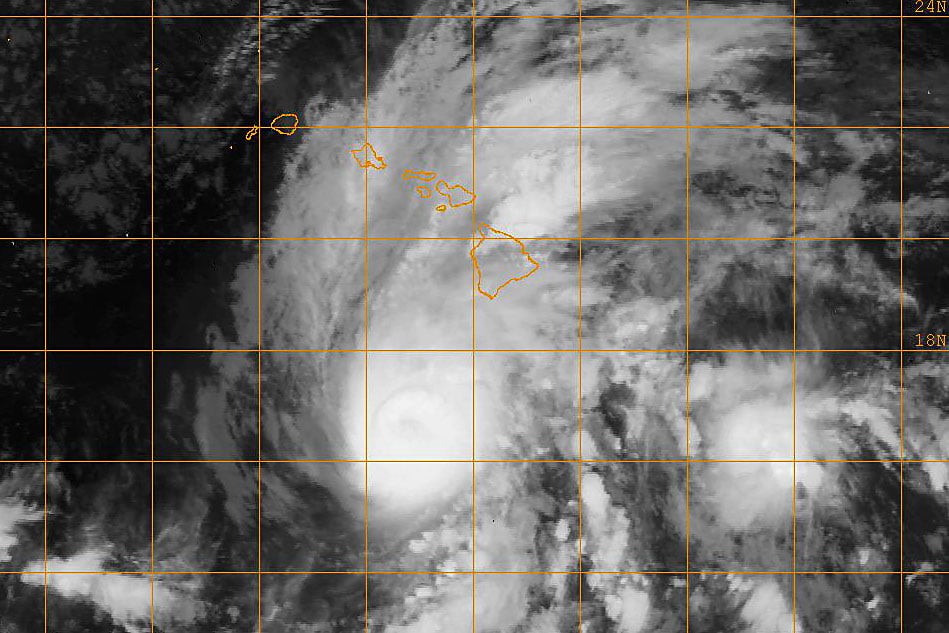This detailed satellite image shows a weather radar focused on the Hawaiian Islands, prominently outlined in orange against a black background that mimics the void of outer space. A distinct orange grid with longitude and latitude markers, including 18N and 24N, overlays the entire rectangular image, providing geographical context. Central to the radar display is a significant weather phenomenon—an expansive tropical storm or hurricane characterized by swirling white clouds. The storm, with its eye beginning to form, is positioned south-southwest of Hawaii, mostly west of the Big Island. The storm's bands extend over about 80% of the Hawaiian Islands, bringing considerable precipitation. Notably, one square on the radar is entirely white, indicating the storm's peak activity. Despite the extensive coverage, the northernmost island, possibly Kauai, remains just outside the storm's immediate influence.